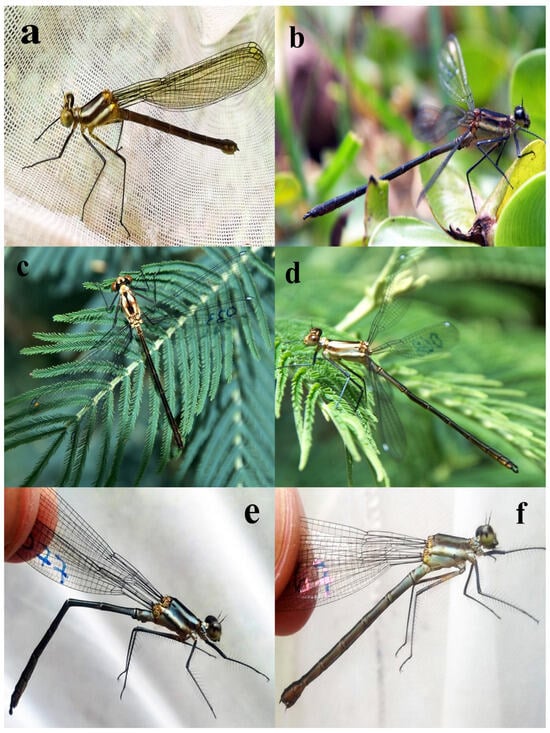This image showcases six meticulously arranged photographs, each depicting a unique insect, specifically dragonflies, labeled from A to F. The photographs are aligned in a 2x3 grid, with two images in each row. 

- **Upper Left (A):** A brown-colored insect, possibly a mosquito or dragonfly, perched delicately, providing a close-up view of its intricate body structure.
- **Upper Right (B):** A vibrant blue dragonfly resting on lush green leaves, highlighting the contrast between its striking coloration and the foliage.
- **Center Left (C):** A dragonfly with a striking black body and gold head, captured in a still pose, emphasizing its unique color combination.
- **Center Right (D):** A stunning, shiny golden dragonfly with translucent wings, elegantly poised on a leaf, showcasing its iridescent beauty.
- **Lower Left (E):** A dragonfly with a black body and clear wings, appearing lifeless as it is held between two fingers. The number "77" is visibly marked on its wing in ink, suggesting it is part of a study or collection.
- **Lower Right (F):** Another dragonfly with a metallic-looking body and translucent wings, similarly held between two fingers by its wings, indicating it may also be part of a scientific examination.

Each photograph provides a detailed perspective of the dragonflies, highlighting their varied colors, delicate wings, and intricate body patterns.